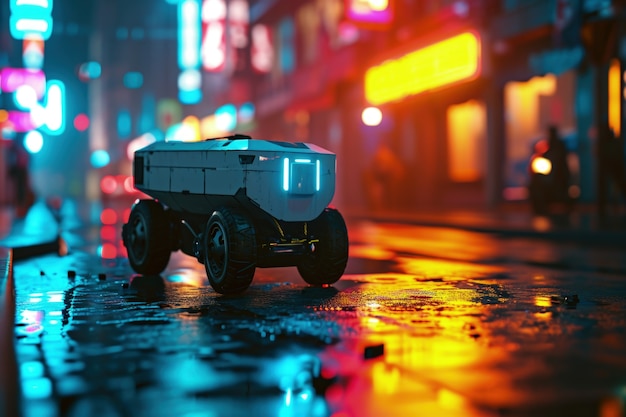The image depicts a vivid nighttime urban scene with a wet road that stretches into the background, illuminated by an array of colorful neon signs. The foreground features a small remote-control vehicle or toy truck with advanced AI or drone-like technology. This vehicle has a sleek white top and four black wheels, with blue neon lights at the front and vertical lights complemented by a horizontal light on top. The road is wet, suggesting it has just rained, and small puddles reflect the glowing neon hues. To the left, a sidewalk runs along the edge, while on the right, blurry figures and store facades add to the bustling ambiance. The neon signs vary in color, with a particularly striking yellowish-golden sign casting a fiery glow on the right side, contrasted by cooler blue and red tones spilling across the left. The overall scene is bathed in bright, saturated colors, creating a dynamic, elemental feel in an otherwise quiet city night.